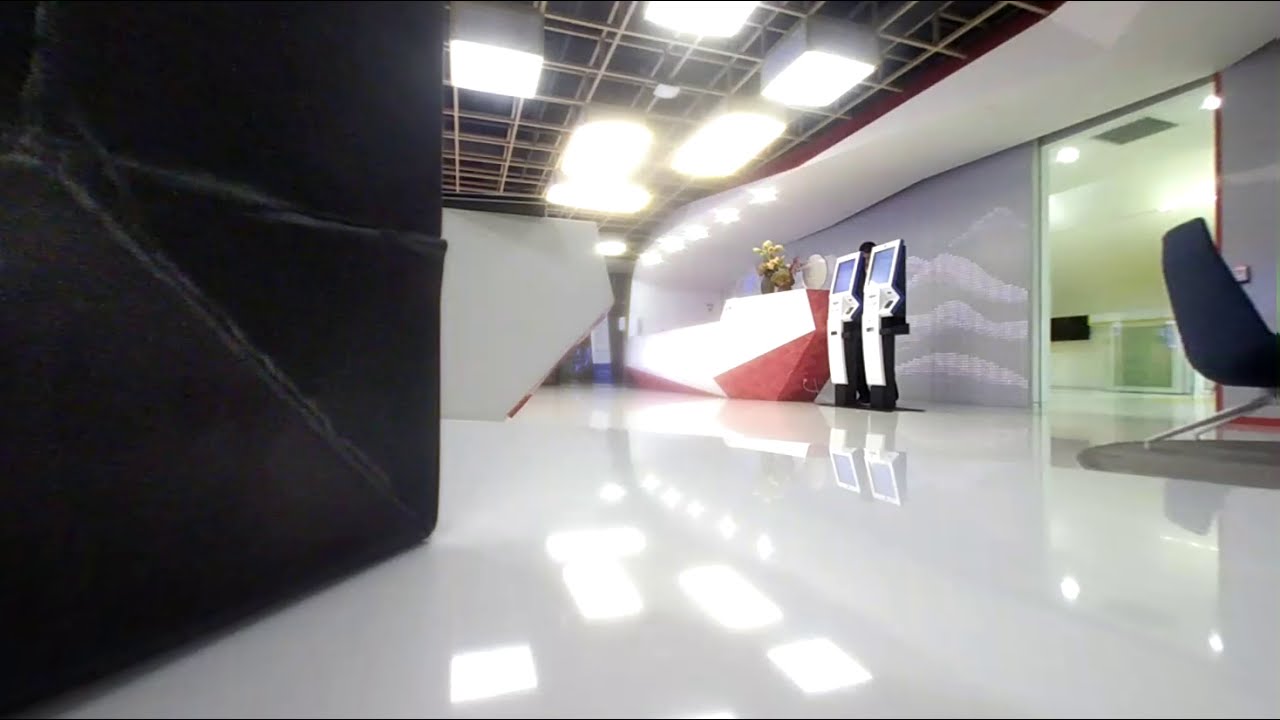The image depicts the interior of a sleek, modern building with a highly polished white floor that reflects the ceiling lights. Central to the scene are two futuristic-looking consoles, characterized by their blue screens and white frames, with their backs appearing black. Adjacent to these consoles is a white entrance desk, decorated with red accents along the bottom and top right corner, and topped by a small green figure resembling a leprechaun wearing a yellow hat. The ceiling above features metal bars and scaffolding, supporting square, gray-cased lights that emit bright white light, which further accentuates the floor's shine. On the far right, a blue high-backed chair with silver rear legs stands next to an open door, revealing an air conditioning unit and a black square object, possibly a towel hanging on a rack. In the far left corner of the image, there is a partially visible black object covered in a crinkled cloth. The setting suggests a commercial or public space with a futuristic aura.